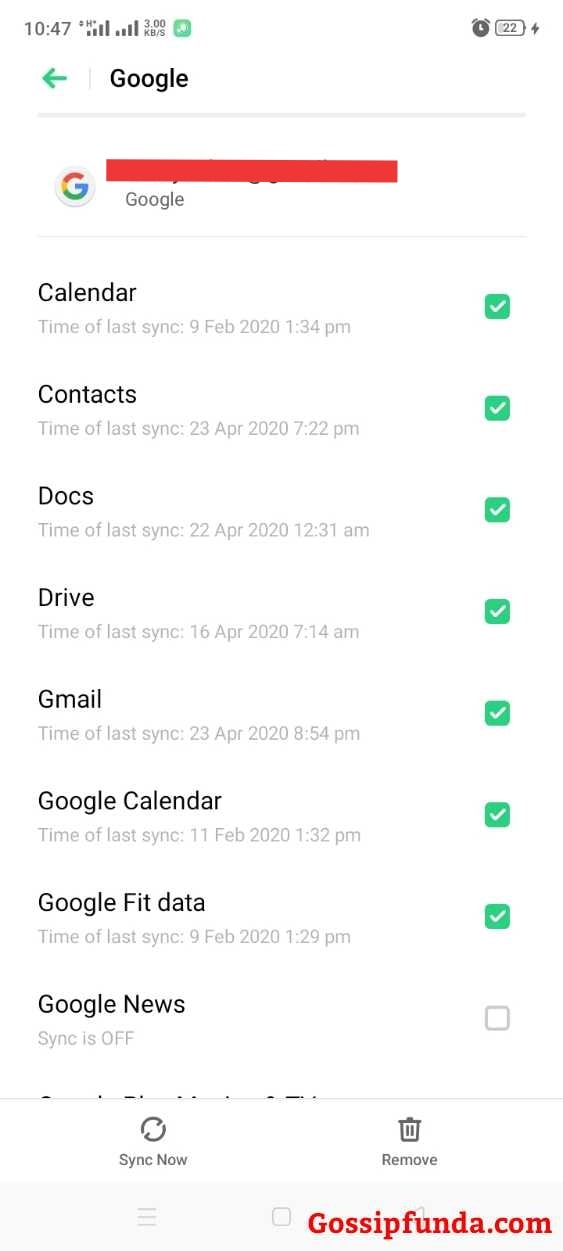This image depicts a synchronization status page on a cell phone with a white background. At the top left corner, the time is displayed as '10:47'. Adjacent to the time are icons indicating cellular connection strength and a square icon with an arrow pointing up and to the right, likely representing 'Upload' or 'Share'. On the far right, there are icons of an alarm clock and a battery indicator.

Just below this top row of icons, the term 'Google' is prominently displayed, accompanied by the 'G' icon for Google. A red bar separates this header section from the rest of the content.

Beneath the red bar, the section begins with 'Calendar', followed by the text: 'Time of last sync: 9 February 2020, 1:34 p.m.' To the right of this text, there is a green square containing a white check mark, indicating successful synchronization.

Next, the same layout repeats for 'Contents', reading: 'Time of last sync: 23 April 2020, 7:22 p.m.' alongside another green square with a white check mark.

The subsequent entries follow a similar format, listing the last sync times for various Google services, each with a corresponding green square and white check mark. These services include:
- Docs
- Drive
- Gmail
- Google Calendar
- Google Fit data

For each of these, the text denotes the last sync time, all accompanied by the green square with a white check mark.

However, under 'Google News', the status indicates that synchronization is turned off. To the right of 'Google News', there's a white box without a check mark, indicating the sync status.

Finally, at the bottom of the page, the text 'gossipfunda.com' is displayed.